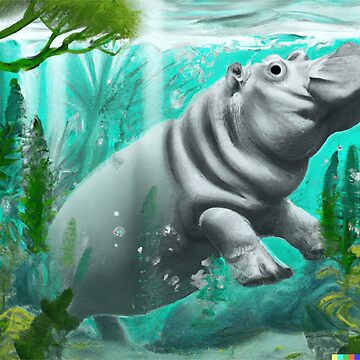This is an illustration, possibly a painting or a computer drawing, depicting a gray hippopotamus underwater in vibrant teal green water. The hippopotamus, with big black eyes and noticeable skin wrinkles, stands on its hind legs, its nose pointed towards the surface, suggesting it is swimming upward. The water appears beautifully tinted with aqua green and some darker gray hues, giving it a sense of depth and wave-like motion. Sunlight filters directly through the water, highlighting the hippopotamus. Surrounding the hippo are numerous plants: green ones behind, to the left, in the front, and even overhead. Some parts of the image, specifically the bottom right, contain blocks of color—yellow, teal, green, red, and blue—adding to the overall vibrant and dynamic underwater scene. Additionally, bubbles are present, enhancing the underwater effect, while the base of the image shows gray tones, possibly depicting underwater soil or further underwater vegetation.